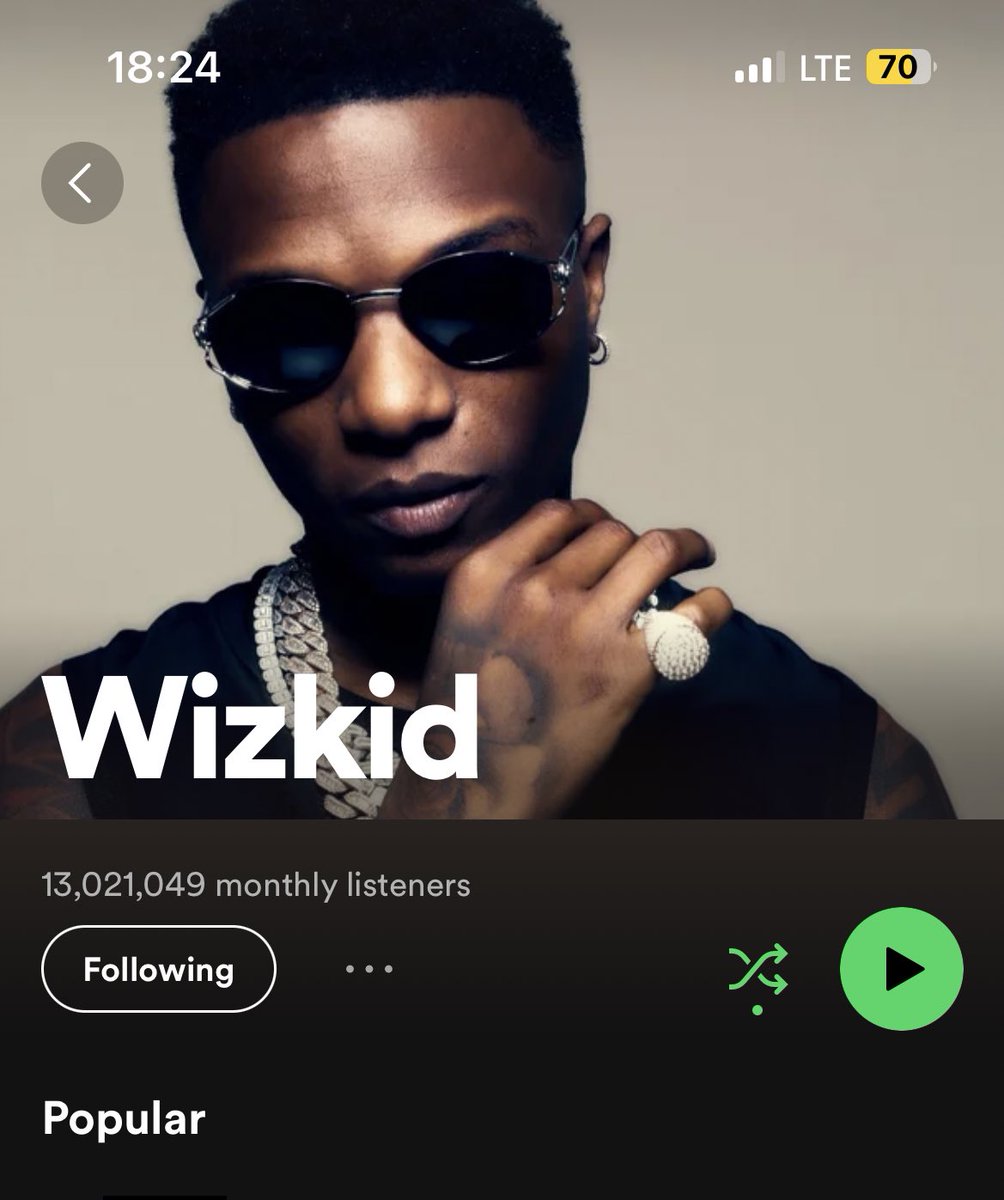The image is a screenshot from the Spotify app, captured on a mobile phone as indicated by the battery icon, data symbol, and time displayed at the top corners. The central focus of the screenshot is the artist Wizkid, whose profile picture is prominently featured in the middle, occupying a significant portion of the image. 

Beneath Wizkid's name, it states that he has 13,021,049 monthly listeners. Below this statistic, there is a white "Following" button, followed by three vertical dots, symbolizing additional options that users can access. To the right of these elements, there are two green icons—one for shuffling music and one for playing. Below the "Following" button, the label "Popular" is visible, suggesting that a list of popular songs would appear if the image were not cut off at that point.

The background of the bottom section of the screenshot is solid black, providing a stark contrast to the detailed header and the artist's image above.